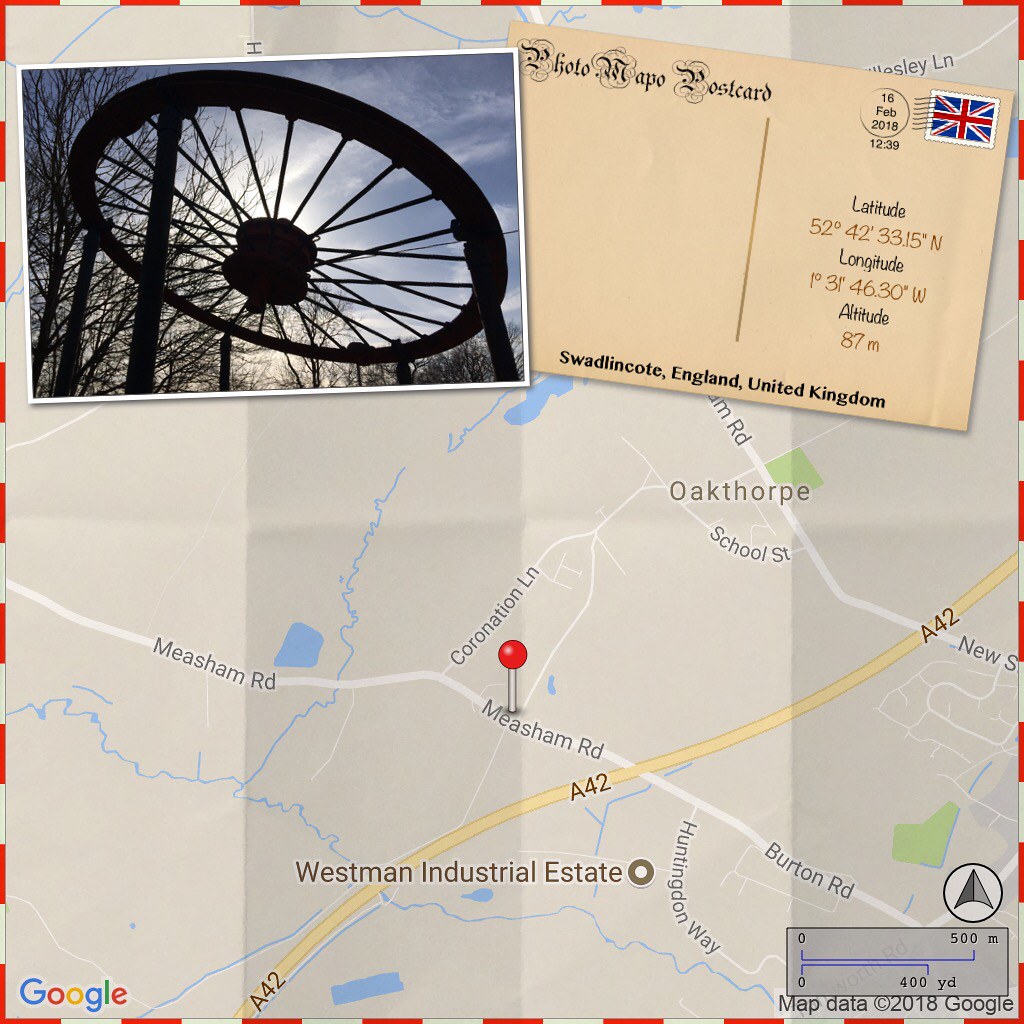The composite image presents a highly detailed visual collage. Dominating the upper left portion, there is a large, horizontally oriented wheel, possibly a fairground ride or swing-supporting structure, resembling an old-fashioned wagon or bicycle wheel, mounted on cylindrical poles. The wheel features a central axle and appears angled, framed by leafless trees against a backdrop of wispy clouds, hinting at a cold day. The sun is partially obscured by the wheel's axle, with the rest of the sky appearing light blue. Beneath this visual, additional foliage is visible.

To the immediate right of the wheel, a sophisticated postcard is prominently displayed. The postcard bears an intricate calligraphy with an illuminated initial letter, and reads "Swadlencote, England, United Kingdom" in a bold mix of upper and lower case letters at the bottom. There’s a British flag postage stamp beside a postmark in the top right corner. Divided vertically, one side of the postcard is reserved for a note and the other for the address. Key geographic coordinates are provided: the latitude is approximately 52.42° N, the longitude 1.31° W, and the altitude 87 meters.

This intricate assemblage overlays a Google map-style background depicting the area around Swadlencote, England. Main roads, such as Misham Road and the A42 freeway, cross the map. Various landmarks like Coronation Lane, Oak Thorpe, School Street, and local parks are clearly marked. The map is segmented into alternating light and dark gray panels and features a legend with a blue line, identifying major routes like Burden Road and Huntington Way. The entire image is bordered by a pattern of red and white hyphens, adding a final touch of detail.

Overall, this image melds a scenic photo, a quaint postcard, and a dynamic map into a rich, historical, and geographical snapshot.